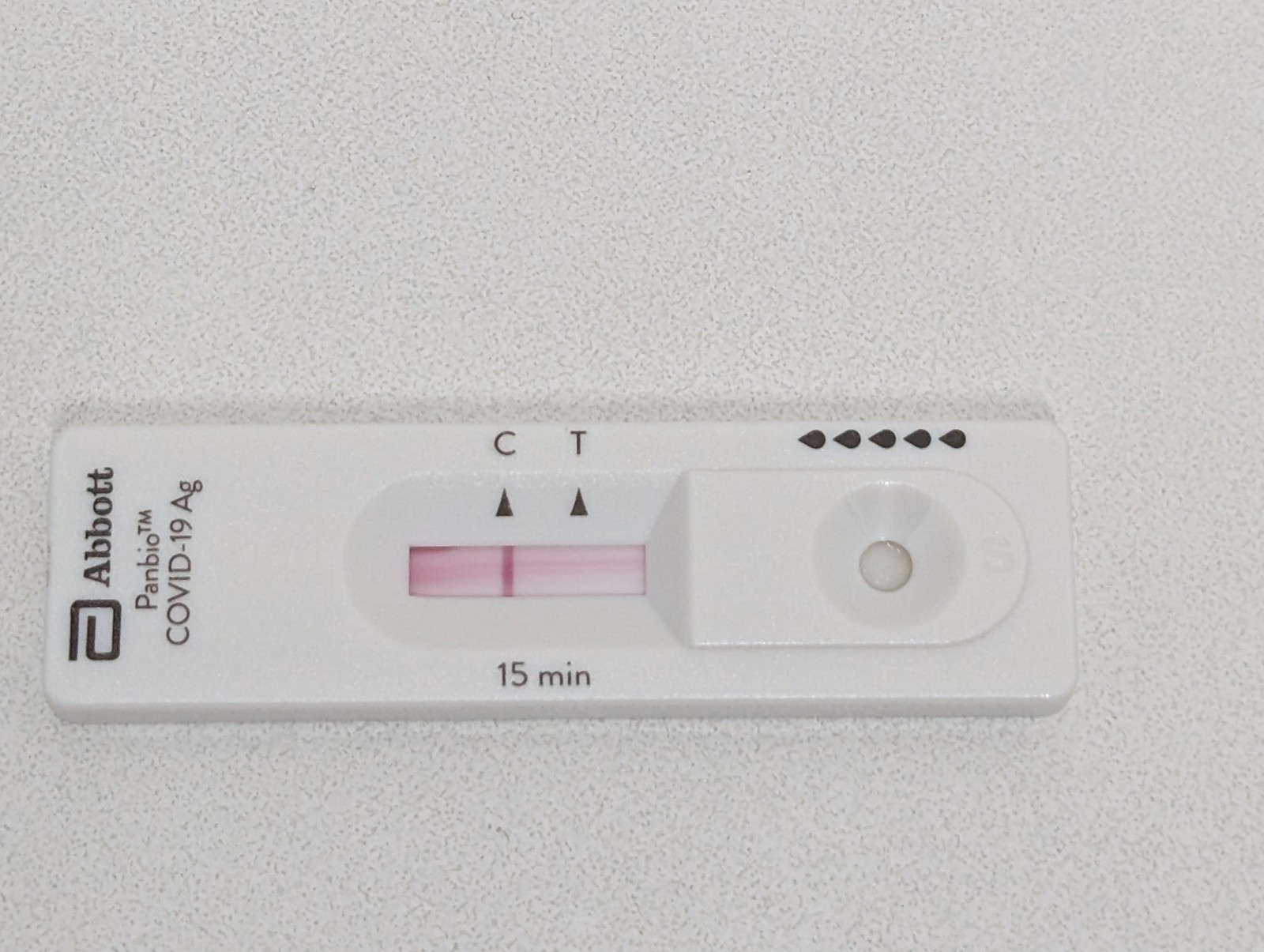This image depicts an Abbott PanBio™ COVID-19 rapid test. The test casing indicates that results can be read in 15 minutes. It features a classic design with 'C' and 'T' markers, where 'C' stands for control. Adjacent to the sample well, there are five small water droplet icons indicating where to apply the liquid sample. The red hue intensifies from the control line towards the top of the test, while the control line itself is clearly marked in red, confirming the test's validity. Below the control line, the front of the test strip is lightly streaked with pink, but notably, there is no visible line at the 'T' marker, indicating a negative result. The entire test apparatus is placed on a surface with gray speckled paper.